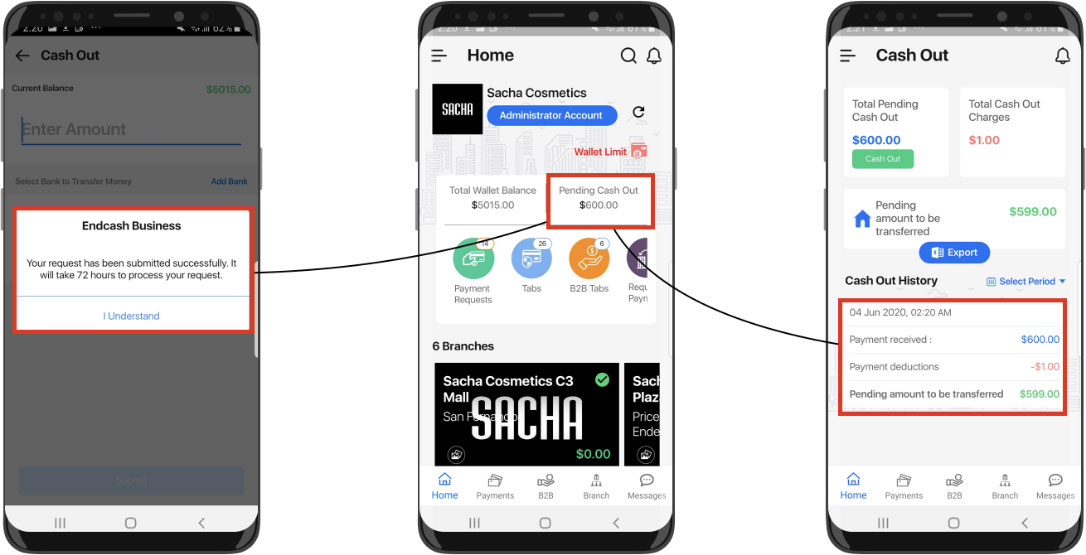This composite illustration consists of three separate images, each displaying a different cell phone screen. 

On the far left, the screen shows a section of a financial application where users can cash out their current balance. The details are somewhat blurry, but there is a visible green dollar amount indicating the balance. It prompts the user to enter an amount, with a red-highlighted box stating "End Cash Business" and a confirmation message: "Your request has been submitted successfully. It will take 72 hours to process your request." Below this message is a clickable "I understand" link.

The central image displays the home page of "Sasha Cosmetics Administrator Account." It includes a wallet limit and various other details. Prominently featured is a red-highlighted square stating "Pending Cash Out: $600," which is connected by a line to the third image.

The third image focuses on the transaction details, displaying "Total Pending Cash Out: $600," "Total Cash Out Charges: $1," and "Pending Amount to be Transferred: $599." There is an export button and another red-highlighted box showing the date and time, "04 June 2020, 2:20 AM." It confirms "Payment received: $600," "Payment deductions: $1," and reiterates the "Pending amount to be transferred: $599." The red-highlighted boxes effectively capture the critical stages and details of the cash transaction process across the three screens.